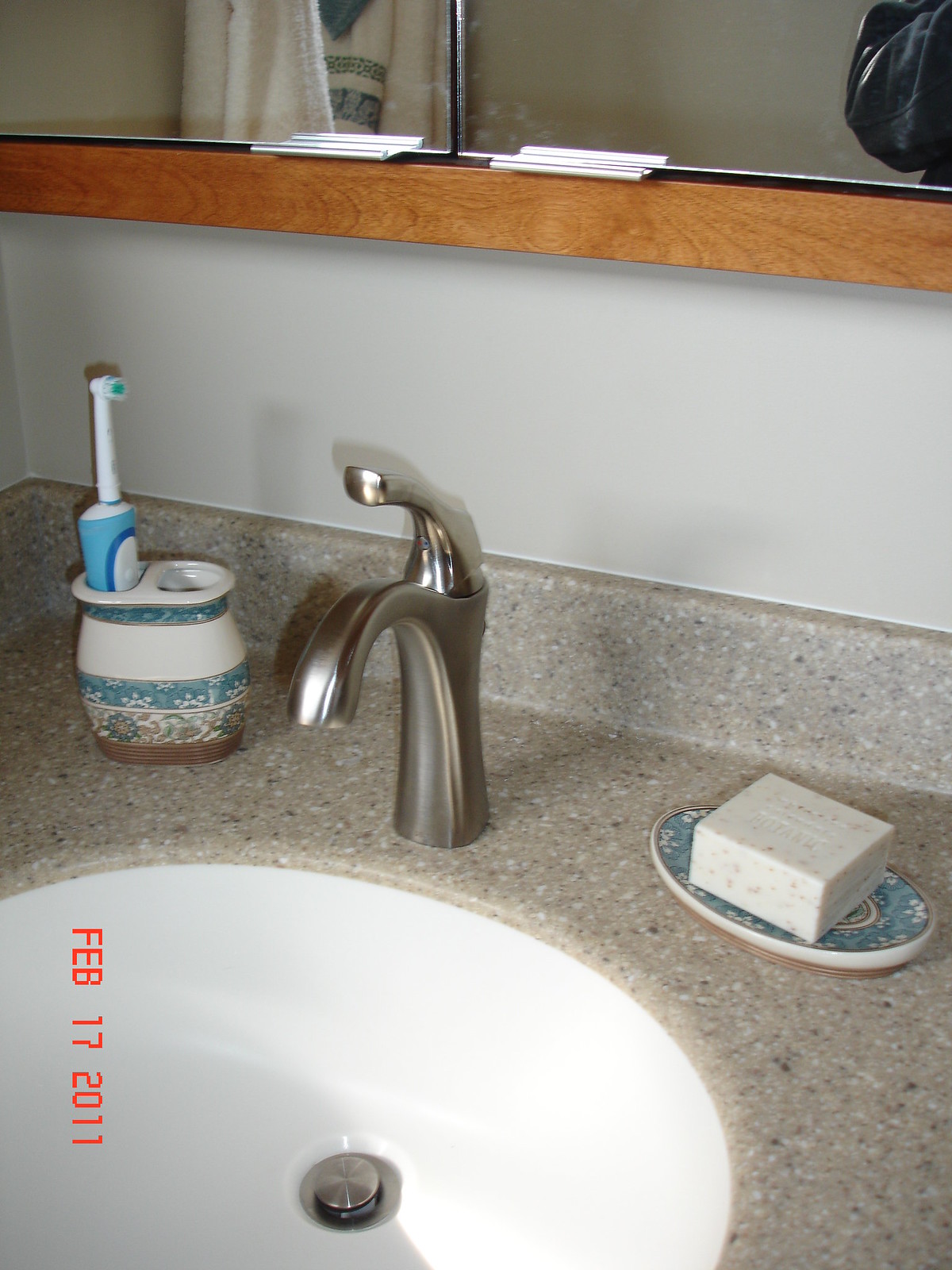The photograph captures a close-up view of a bathroom sink. The countertop features a light brown surface adorned with black and white speckles, resembling a granite pattern. The sink basin itself is a pristine, shiny white, complemented by a silver faucet. Positioned to the right of the faucet is a blue soap dish holding a square bar of soap. On the left side of the faucet sits a toothbrush holder with a white and blue floral pattern. The holder has two slots; the left one contains a toothbrush with a round head, while the right slot remains empty. Mounted on the wall above the sink is a medicine cabinet with two mirrored doors, each equipped with small silver handles at the bottom. The cabinet is framed with brown wood. Notably, the photograph has a timestamp reading "Feb 17, 2011" vertically along the bottom right-hand side, indicating the date the photo was taken.